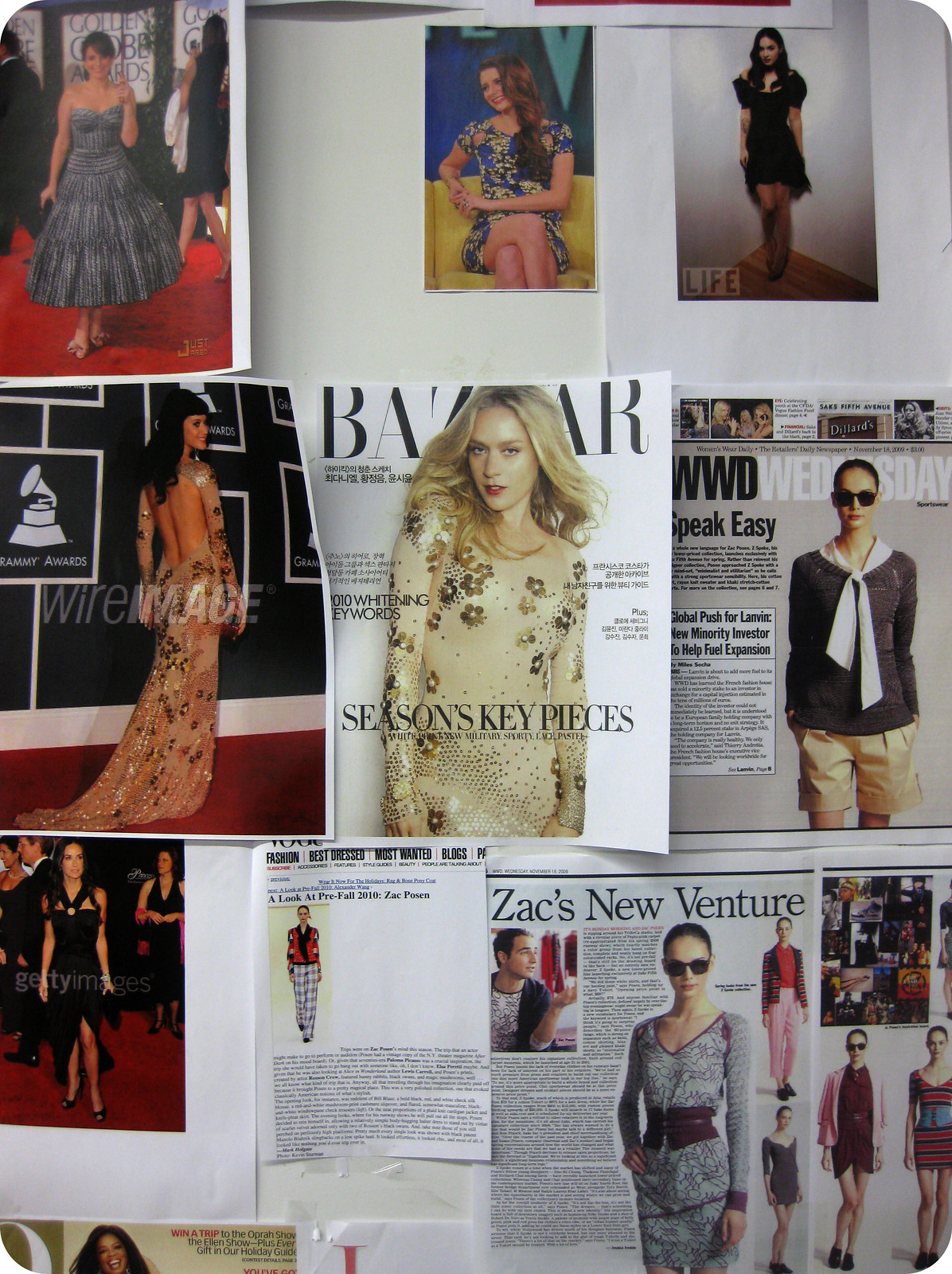This image is a vertically aligned, rounded-corner rectangular collage featuring an array of fashion magazine clippings and photocopies, all taped to a white wall. In the very center, a Bazaar magazine cover showcases a blonde model in a long, multicolored dress, with the text "Seasons Key Pieces" prominently displayed. Adjacent to this, an insert labeled "WWD Wednesday" presents a woman in a black sweater, white scarf, and khaki shorts.

In the upper left, a woman with brown hair is pictured on the red carpet, wearing a sleeveless dark gray ruffled dress. To her right, another image shows a woman in a blue and yellow floral dress, sitting on a yellow sofa. Further right, a smaller clipping from Life Magazine features a woman with long dark hair in a black dress, exuding a mysterious aura.

The bottom left of the collage contains another red carpet photograph of a woman in a long backless golden gown, marked with the text "Wire Image." Beside this is a printout with predominantly white text and a small image of a woman in plaid pants and a red and black top. The lower right corner features a newspaper clipping titled "Zach's New Venture," depicting several people.

Across the collage, there are additional images of women in various dresses and outfits, contributing to a vibrant medley of fashion styles and poses. This eclectic assortment emphasizes the diversity and creativity of contemporary women's fashion.